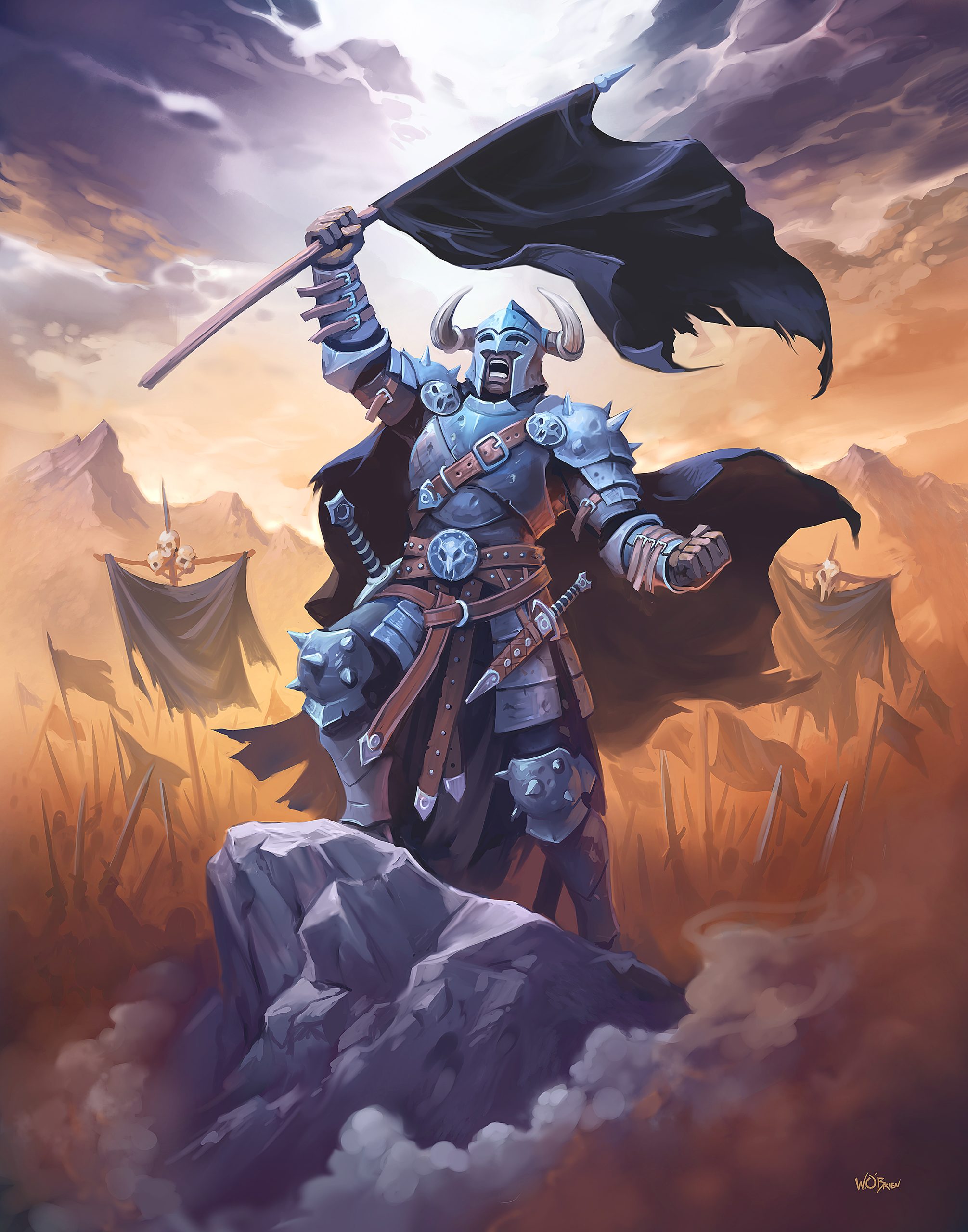The image is an intense and vividly detailed war scene, possibly from a poster, comic book, or a graphic art piece. It features a Viking-like warrior clad in full silver body armor, complete with a helmet adorned with bull-like horns. The warrior stands defiantly on a rocky cliff, his right hand raised high, clutching a slightly torn black flag with a spear pole. His mouth is open in a victorious scream directed towards the dramatic, overcast sky that is tinged with a hint of sunlight breaking through. The warrior also sports a cape flowing behind him, a sword sheathed at his belt, and a dagger on the other side. Surrounding him are ominous stakes topped with human skulls and black flags, adding to the grim atmosphere of the scene. The background hints at chaos, with elements that suggest it might be ablaze. There is a signature in the bottom right corner, marking the artist's identity.